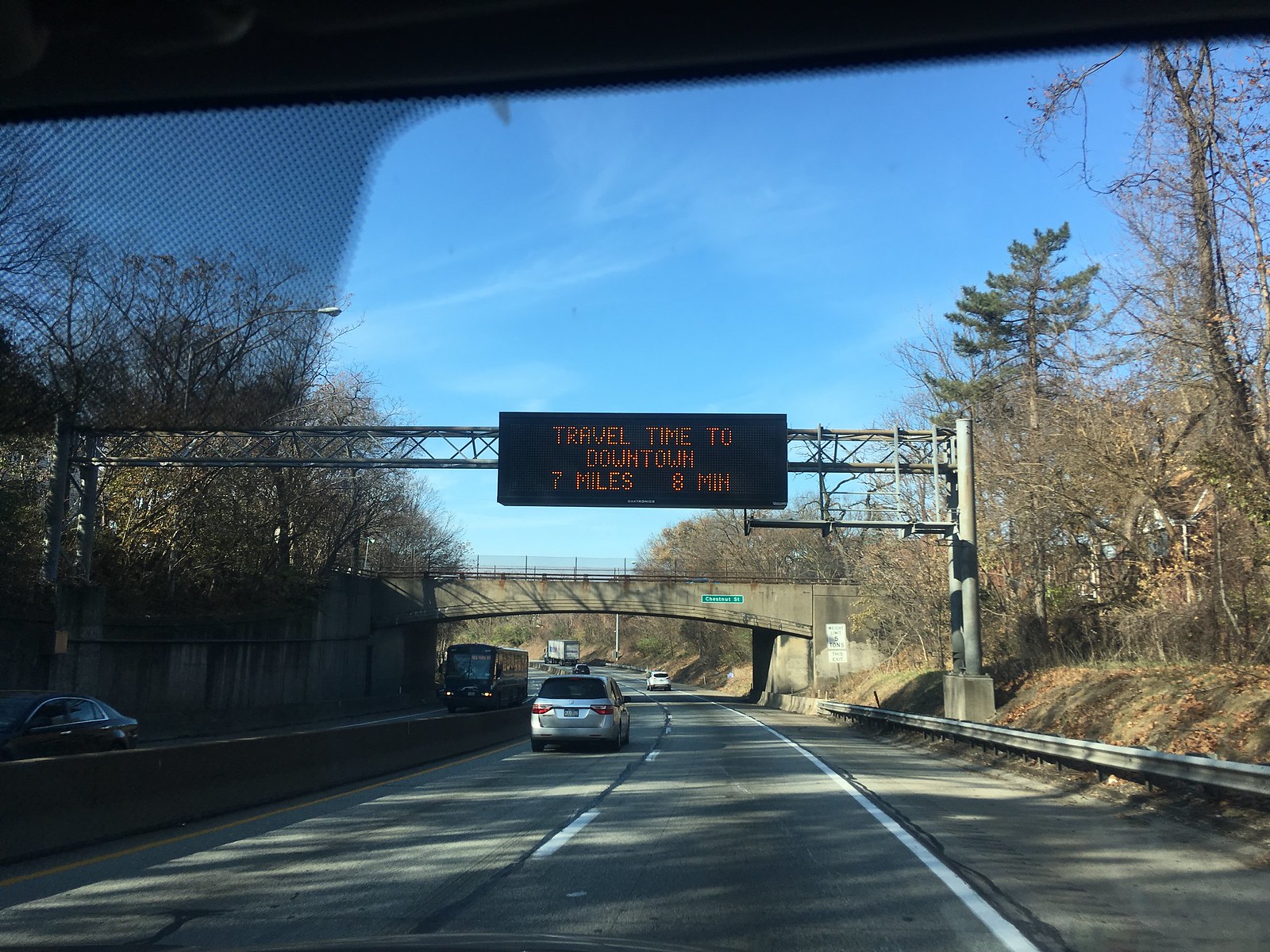The image captures a two-lane expressway, photographed from inside a car traveling in the right lane. The highway features a concrete barrier dividing the lanes heading in opposite directions. Overhead, there's a black digital sign with orange pixelated text indicating "Travel time to downtown: 7 miles, 8 minutes." Surrounding the road, both to the right and left, are numerous leafless trees, hinting it is either late fall or early spring, under a blue sky with light clouds. Various vehicles populate the scene, including a silver car directly ahead in the left lane, and in the distance, a truck by the roadside and a black bus crossing a median. Steel beams line the roadside to the right, protecting cars from veering off into nearby hills dotted with trees. The left-hand side of the image subtly features the pixelated dots of a windshield visor, confirming the photo’s in-car perspective. The familiarity of the scene suggests it could be an urban highway, possibly reminiscent of cities like Chicago.